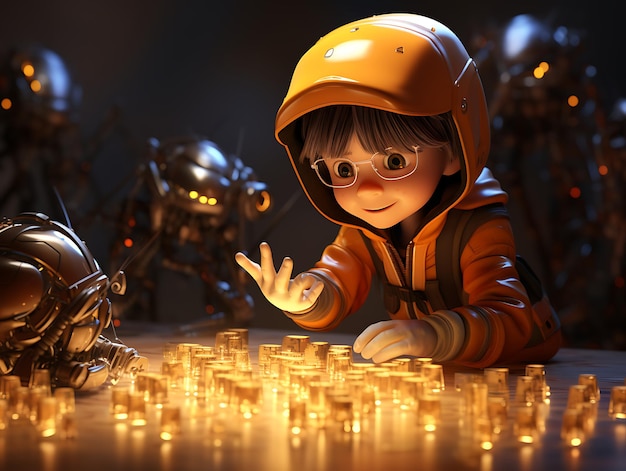In this highly detailed, high-resolution 3D digital art, a young boy with brown hair and eyes, wearing white glasses, is depicted. He is dressed in an orange jumpsuit and helmet, and is crouched or perched on the ground, propped up on one elbow. The child appears engrossed in examining several small, translucent cubes scattered on the floor in front of him, all glowing with a yellowish-gold light. Surrounding the boy are several small, dark gray robots, three of which are in the background and one positioned in the foreground to the left. The boy's left hand is making an OK symbol towards the robot on the left. The scene is intricate and radiates a sense of curious engagement between the boy and the mechanical companions.